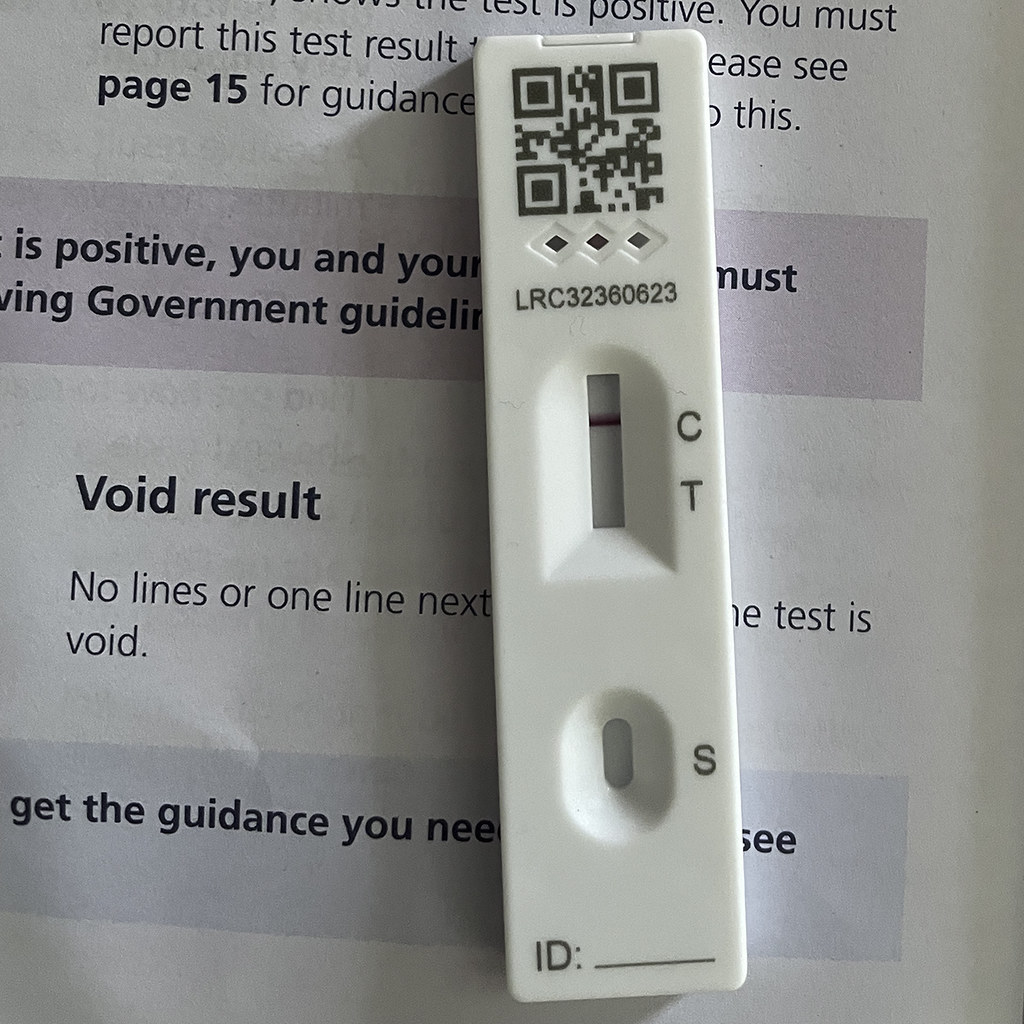This photograph features a plastic test kit with various indicators and labels designed for a specific type of diagnostic test. The test kit is housed in a white plastic casing.

At the top of the test, there is a QR code for scanning purposes. Directly below the QR code, the casing is adorned with rows of black, sideways-facing diamonds. Further down, there is an inscription that reads "LRC 32360623."

Below this inscription, there is an indicator window. Beside the letter "C" on the right side of the indicator window, there is a single red line, signifying a specific result. Notably, there is no line next to the letter "T," which is positioned below the letter "C." This suggests the test results are negative. 

Further down, there is another separate indicator window marked with the letter "S," although this window does not display any visible lines or markings.

At the very bottom of the test, there is a field labeled "ID:" followed by a blank space provided for writing the ID number, though it currently remains empty.

The test device is resting on top of an accompanying pamphlet. The pamphlet appears to offer instructions and details regarding test results, including information about a "void" result if "no lines" or "one line" is visible in certain positions. However, part of the text is obscured by the test device itself. The pamphlet also references government guidelines for reporting the test results.